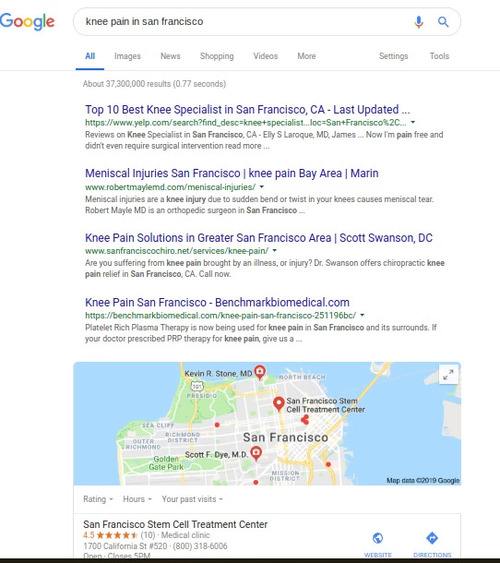Screenshot of a Google search page with the query "knee pain in San Francisco" showing four search results. 

1. **First link**: "Top 10 Best Knee Specialists in San Francisco" from Yelp.com.
2. **Second link**: "Meniscal Injuries: San Francisco Knee Pain Bay Area Marin" from RobertMayford.com.
3. **Third link**: "Knee Pain Solutions in Greater San Francisco Area" from SanFranciscoCairo.net.
4. **Fourth link**: "Knee Pain San Francisco" from BenchmarkBiomedical.com.

Below the search results, there is a map of San Francisco featuring red location bubbles indicating the offices of the knee specialists. Underneath the map, four tabs labeled "Ratings," "Hours," "Your Past Visits," and "More" are present. 

The detailed information from the "Ratings" tab includes:
- **San Francisco Stem Cell Treatment**: 
  - **Rating**: 4.5 stars, based on 10 ratings.
  - **Address**: 1700 California Street, Suite 520.
  - **Contact**: Includes a phone number and clickable icons for the website and directions located on the far right side.